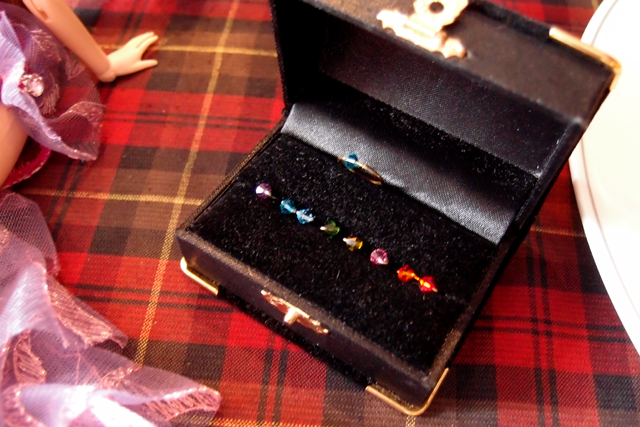In this photograph, a small black jewelry box is showcased against a vivid red tartan plaid, which features prominent black squares intersected by intricate yellow lines. The jewelry box, lined with luxurious black velvet, is open, revealing its plush, cut-to-fit black interior that securely holds an array of precious stones. Highlighting the box's design, gold bands adorn the corners of both the lid and base, and a gold latch is prominently displayed at the top.

Inside the box, a collection of multicolored jewels is meticulously arranged in horizontal rows, including pink, blue, gold, and red stones. Additionally, a golden ring set with a striking blue gem is slightly off-center to the left, nestled within the elegant interior.

To the right side of the image, the red fabric curves gracefully in an arc, while to the left, the partial figure of a doll is visible. The doll, dressed in a purple outfit with glittering tulle or lace, extends her left arm into the frame, contributing to the whimsical quality of the scene.